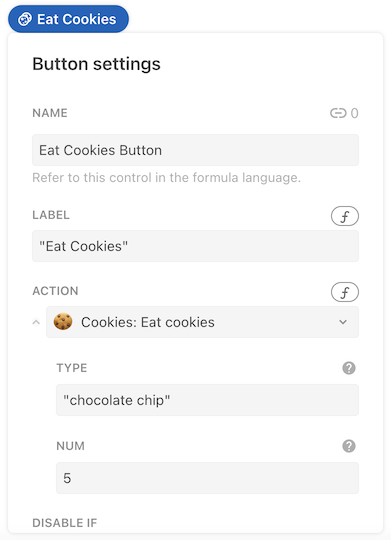"A digital screenshot presenting a cookie notification interface is shown at the top left corner. The interface features a prominent blue and white button labeled 'Eat Cookies' alongside two small images of cookies. 

Adjacent to this button, there is a Settings option, allowing users to manage cookie preferences. A label option also appears on the interface, displaying the text 'Eat Cookies' in quotes. 

Directly below, a lowercase 'f' is visible, followed by the word 'Action.' The recurring phrase 'Cookies: Eat Cookies' is highlighted, emphasizing the action associated with the button.

Additionally, a small chocolate chip cookie image is displayed. The cookie is tan in color, adorned with a total of six chocolate chips. Below this image, the type is specified as 'chocolate chip' in quotes. Finally, the word 'NUM' is presented, with the numeral five indicated below it."